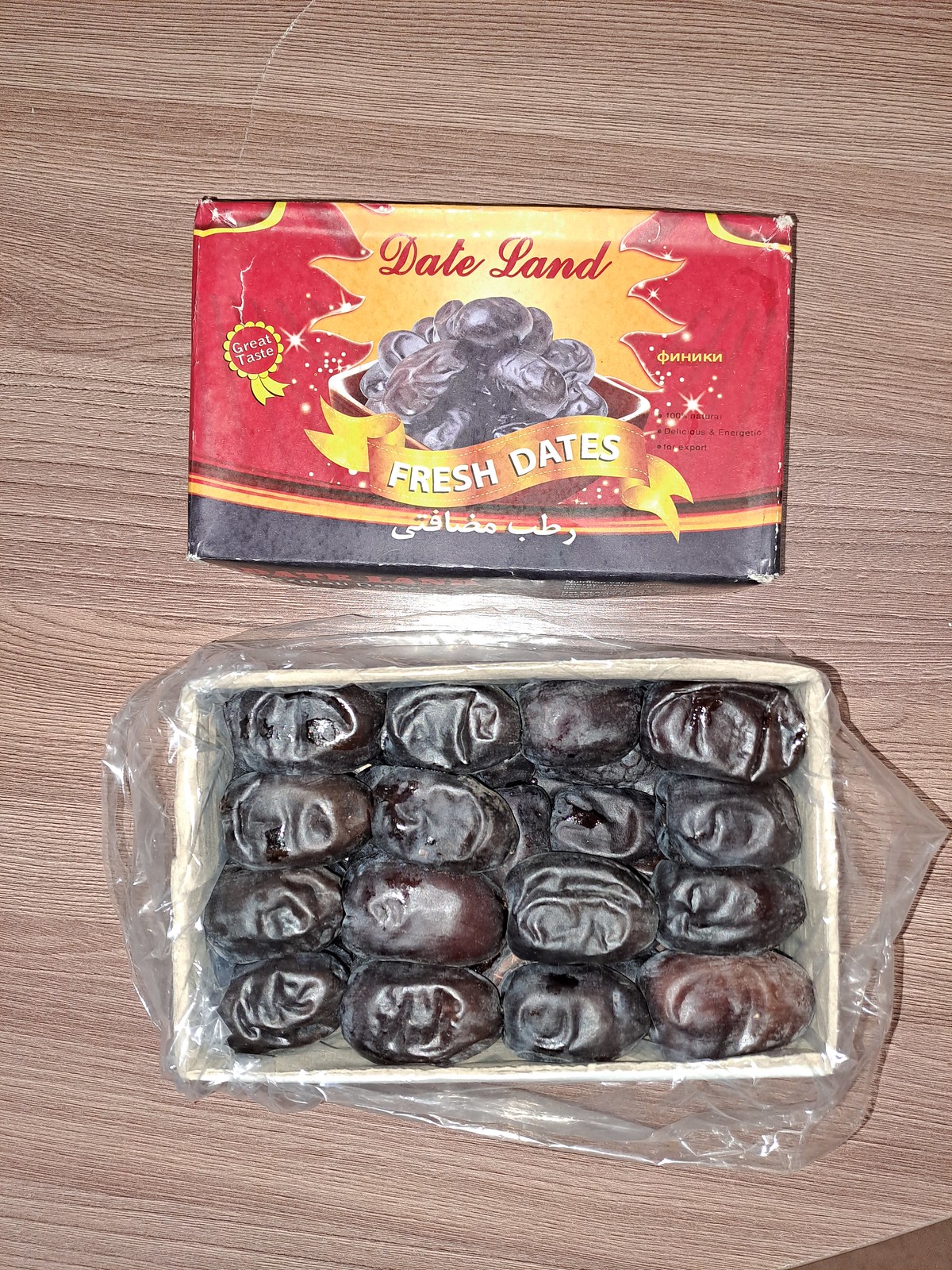The image showcases a package of fresh dates on a light brown wooden table. The packaging, which is rectangular and has been placed atop the container, features a red background with a gold starburst at the top that says "Date Land" in red script. To the left side of the red packaging, there is a ribbon-shaped design with a circle surrounded by petal-like shapes and ribbons hanging from it, stating "Great Taste" in white text. An orange ribbon also displays "Fresh Dates" in white font. Additionally, the right side of the packaging includes yellow Russian text and the phrases "100% natural," "Delicious," and "Energizing" in black and white lettering, some of which are partially obscured by white stars. The dates themselves, visible through a clear plastic wrap, are arranged in a white rectangular container and display varying shades of dark purple with a slightly wrinkled and shiny appearance.